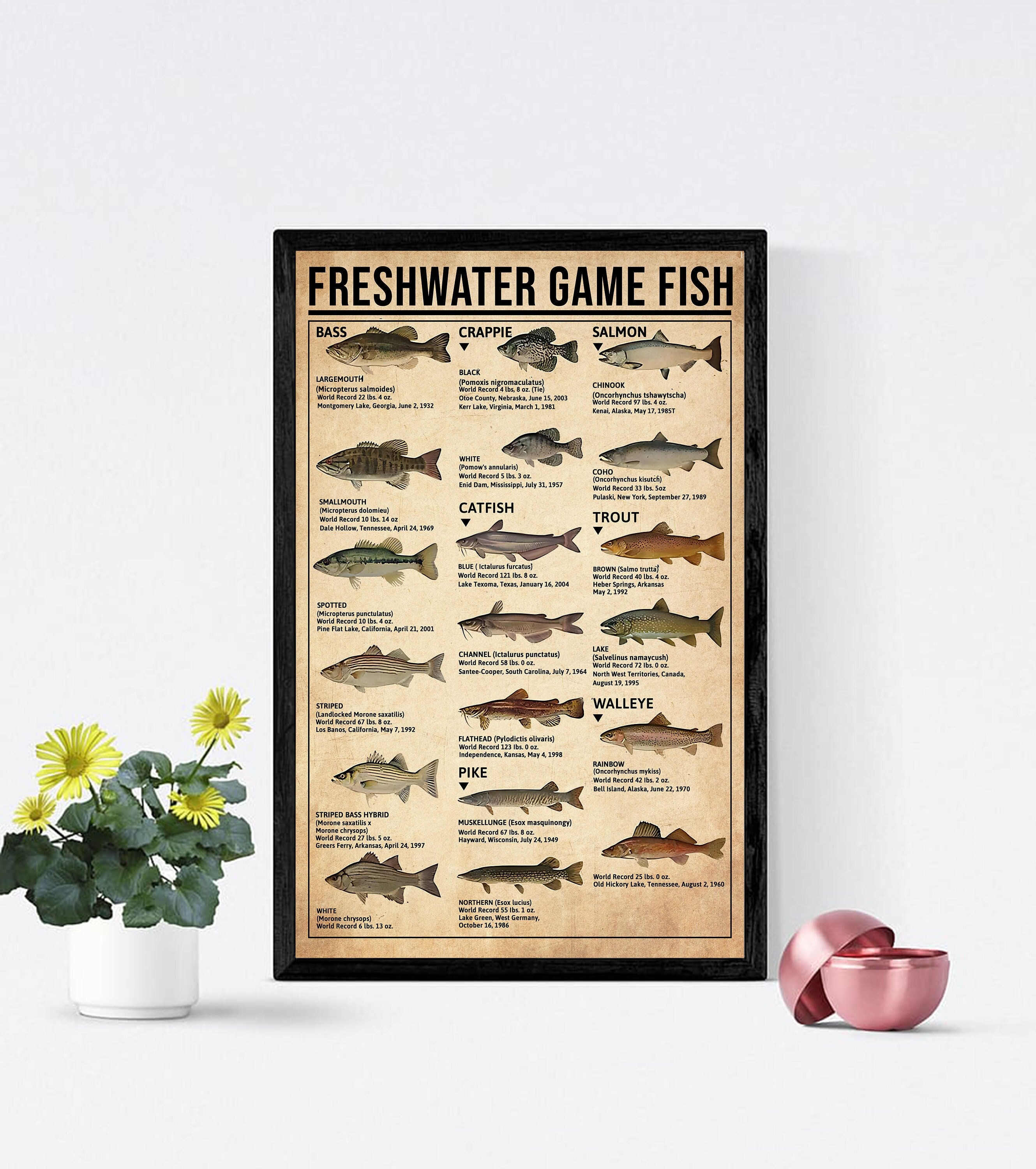The image features a professionally edited product photograph showcasing a rectangular poster set against a flat, white background. Designed for commercial purposes like online shops or catalogs, the poster is framed in sleek black wood and exhibits a light brown background. At the top of the poster, in bold black font, reads "Freshwater Game Fish." The poster meticulously illustrates various freshwater fish, including easily identifiable types such as bass, crappie, salmon, carp, catfish, trout, walleye, and pike. These fish are arranged in a structured format of three columns and six rows, with individual tags listing their names. Some text is smaller and less legible, offering additional details of the fish. Alongside the framed poster, props include a potted yellow flower on the left and an empty, open silver capsule on the right, adding visual interest to the minimalist setup.